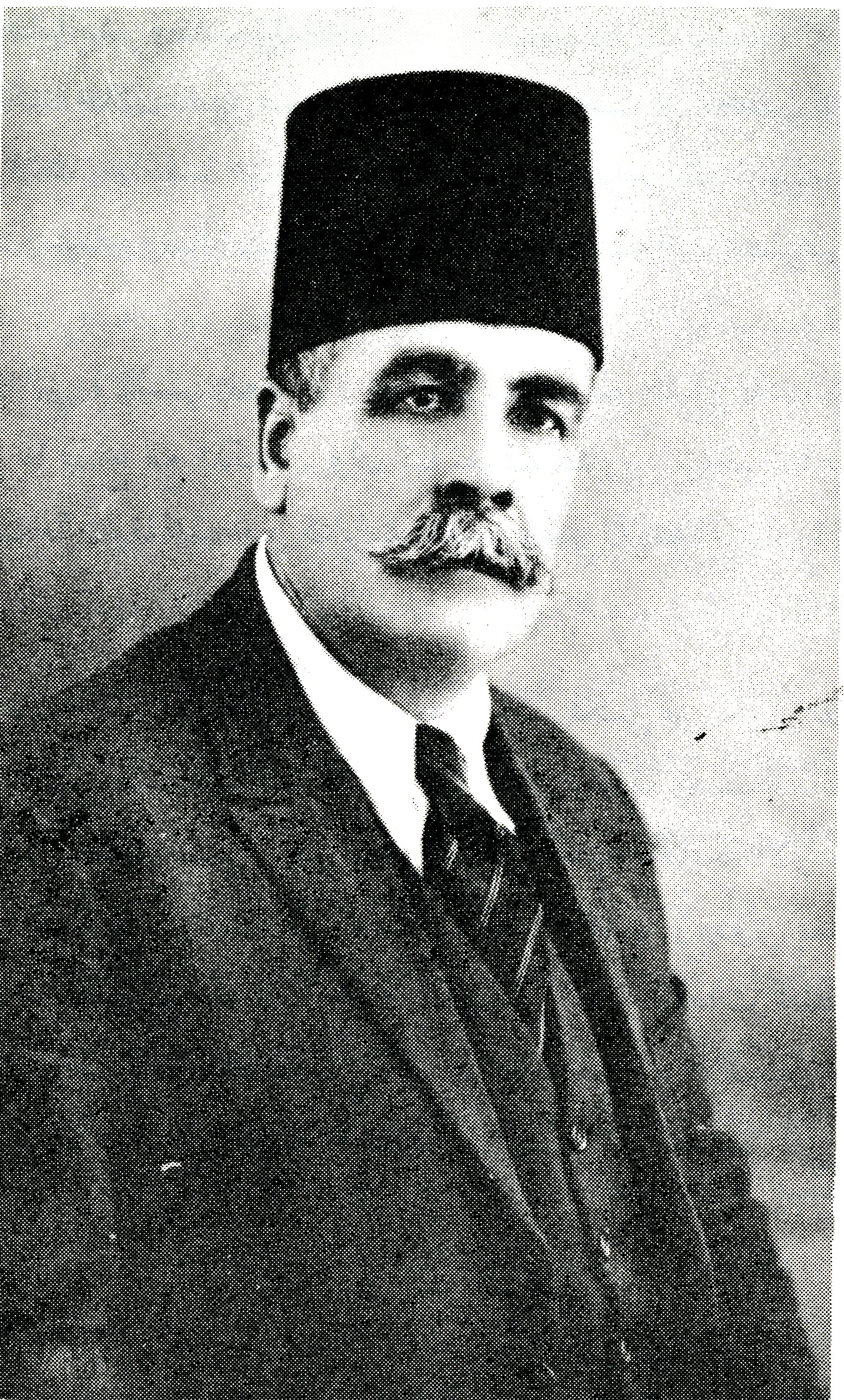This is a black and white photograph of an older gentleman wearing a distinctive black cap that resembles a Shriner's fez, but without any tassel or ornamentation. He has a substantial, graying mustache that extends around the corners of his mouth and bushy eyebrows. Wisps of graying hair are visible peeking out over his right ear from beneath the hat. The man is dressed in a polished three-piece suit: a dark jacket, a matching dark vest, and a white shirt accented by a dark tie with lighter diagonal stripes. He looks directly at the camera with an expression that suggests a posed portrait, possibly from the early 1900s. The background of the photo is plain white, and there is no text or lettering on the image. Shadows, especially around his right eye, add depth to his features, highlighting his pronounced facial characteristics.